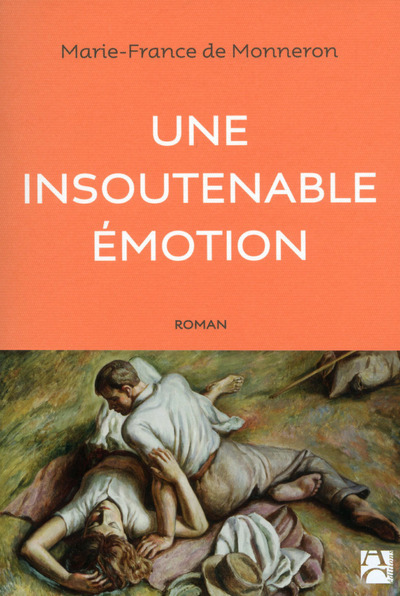This cover image features a French book titled "Une Insoutenable Emotion" by Marie-France de Monneron. The top portion of the image presents an orange background with the author's name, "Marie-France de Monneron," written in black serif font, followed by the book title in white, all caps sans serif font. Below the title, the word "Roman" appears in small black letters. 

The bottom half of the cover showcases a colorful painting of a man and woman on the ground. The woman, with long wavy red hair, is reclined on what appears to be a blanket, her eyes closed and her left hand above her head. The man, who has short blonde hair, is sitting beside her, leaning over and propping himself up with his left arm, gazing at her with a tender expression. Scattered around them are a hat and several articles of clothing, suggesting an intimate, relaxed setting. The backdrop has an impressionist quality, enhancing the romantic and serene atmosphere. In the bottom right-hand corner, the letters "AC" are visible, indicating the publisher or edition. The overall scene is brightly lit by natural light, making the details clear and the mood inviting.